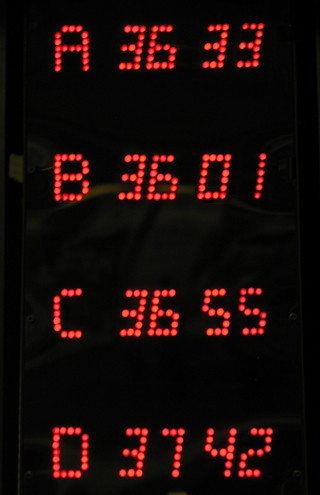The image is a photograph of a black LCD screen displaying red digital characters. Each line on the screen presents a letter followed by a two-part number, separated by spaces. The top line reads "A 36 33," where "A" is followed by the number "36.33." The second line reads "B 36 01," the third reads "C 36 55," and the fourth reads "D 37 42." The characters are made up of glowing red dots, suggesting a digital display. This could indicate scores, measurements, or timings, potentially for a competition. The context hints at results such as times for runners or swimmers, with "36" likely representing seconds and the subsequent digits representing milliseconds.